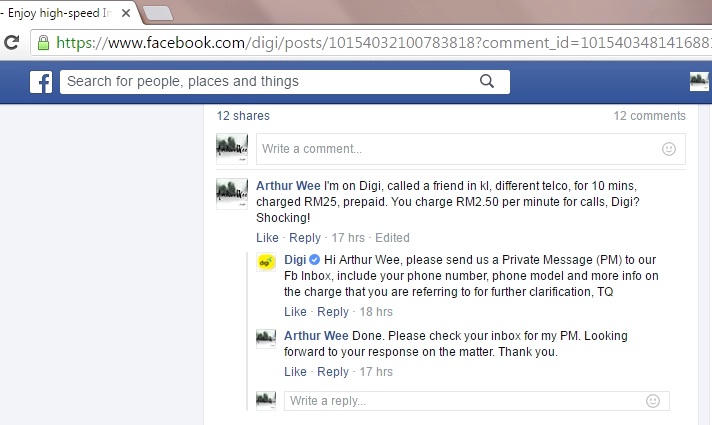This detailed color image is a screenshot of a computer screen displaying a Facebook page. The web browser shows a single open tab with the text "Enjoy High Speed," partially cut off, along with the URL: https://www.facebook.com/digi/posts. The familiar blue Facebook banner is visible at the top, featuring a white Facebook logo within a blue box and a search bar labeled "Search for people, places, and things."

Beneath the banner, the screen displays a post from Arthur Wee. Arthur Wee, who is using the Digi telecom service, comments that he called a friend in Kuala Lumpur (KL) who uses a different telecom service. He mentions that he was charged RM 25 for a 10-minute prepaid call, while Digi charges RM 2.50 per minute, expressing his shock at the high rate: "I'm on Digi, called a friend in KL, different telco, for 10 minutes, charged RM 25 prepaid, you charge RM 2.50 per minute for calls, Digi? Shocking!" 

In response to Arthur Wee's complaint, Digi replies, "Hi Arthur Wee, please send us a private message to our Facebook inbox, include your phone number, phone model, and more info on the charge that you are referring to for further clarification, TQ." Arthur Wee confirms his compliance in his follow-up comment: "Done, please check your inbox for my PM, looking forward to your response on the matter, thank you." 

The image further shows that the post by Arthur Wee has garnered 12 shares and presents a section to write comments, indicating engagement from other users. This screenshot highlights a customer attempting to resolve a billing issue directly through the company's Facebook page, illustrating the modern use of social media for consumer queries and company responses.